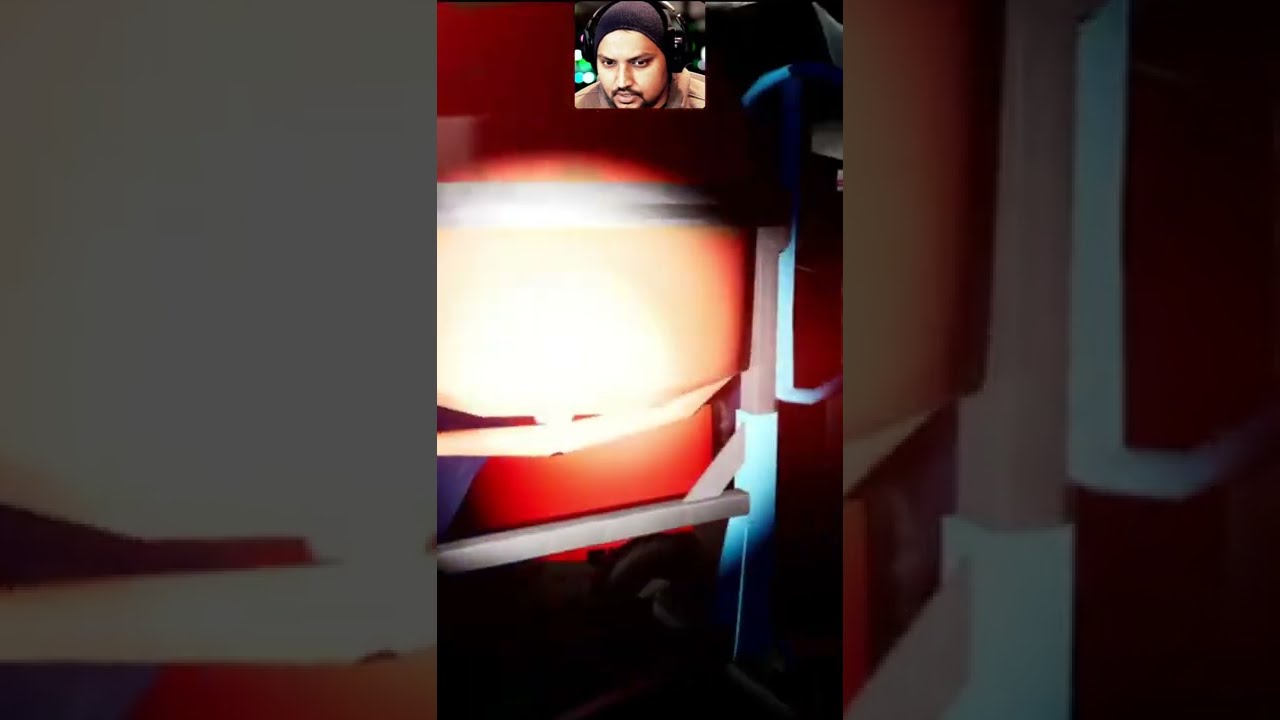The image is a blend of vibrant and subdued colors divided into three sections: left, center, and right. The central panel, which is the main focus, features a close-up of a man's face wearing headphones and a black toboggan or cap. His face, illuminated by a flashlight, reveals dark olive skin and a slight mustache and beard. The man's intense gaze is directed forward, and he is framed by an orange tank with portions in shadow, suggesting it might be in a dark room with isolated areas of bright light. Surrounding the man, there are fragments of cream, light blue, and red colors, with the left and right panels possibly being close-up versions of the central image. The right panel includes some white horizontal and vertical beams that form an L shape and contrasts sharply with the darker surroundings, giving the scene a somewhat blurry and difficult-to-discern composition.